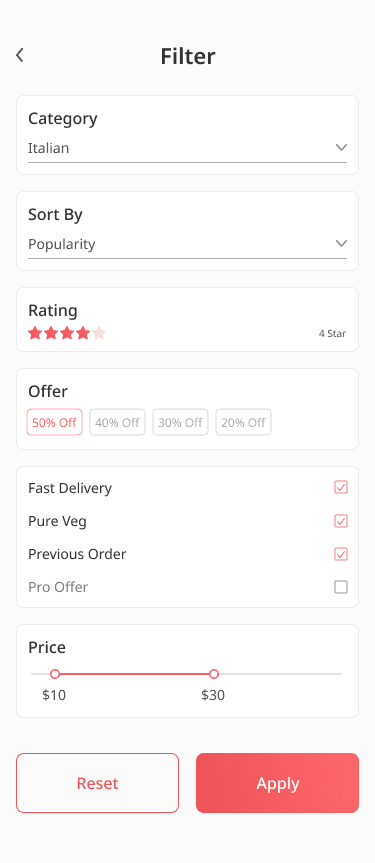The image presents a well-structured, colorful interface divided into multiple sections, each distinguished by unique colors, shapes, and sizes. These subsections categorize different topics, enabling users to easily locate specific information. Scattered across the top, middle, and bottom of the image are various symbols that provide additional details or functionalities when accessed. The majority of the text is in black, featuring varied font sizes and styles for emphasis and readability. The overall layout is straightforward and user-friendly, ensuring accessibility with minimal to no difficulty for any user.